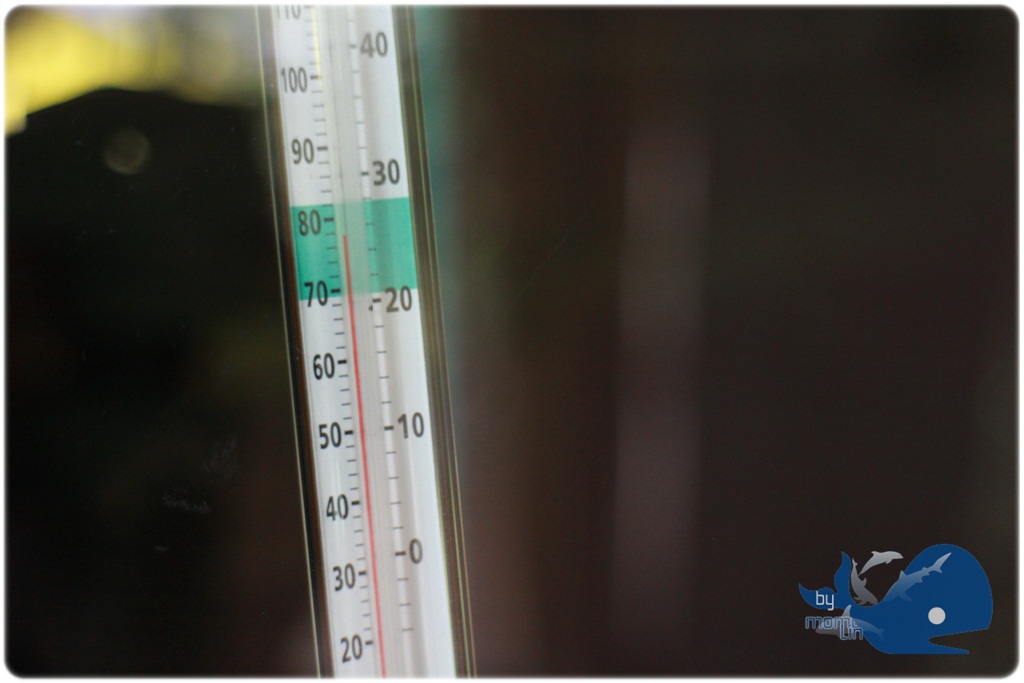This horizontal rectangular photograph features a vertically oriented thermometer prominently displayed slightly left of center. The thermometer extends from the top almost to the bottom of the frame, although the top and bottom are cut off, making it not fully visible. 

The thermometer is predominantly white with numerical markings on both sides indicating temperature values. On the left side, the visible numbers descending from top to bottom are 100, 90, 80, 70, 60, 50, 40, 30, and 20. The bottom-most number visible is 20. The right side of the thermometer shows numbers descending in reverse order: negative 40, negative 30, negative 20, negative 10, and zero. Each of these major numbers is accompanied by smaller horizontal lines marking incremental values.

Near the center of the thermometer, there's a shaded green section that spans just below the 70 mark to just above the 80 mark, indicating a specific temperature range. A red vertical line within the thermometer runs from just below 80 towards the bottom edge of the image, where it is cut off.

In the bottom right corner of the photograph, there's a small cartoon featuring a dark blue whale with a white eye. Additional gray marine creatures, potentially dolphins or sharks, appear to be swimming around the whale. Above the whale, there are the white letters "by" in lowercase, followed by an illegible name.

The surroundings of the thermometer are predominantly dark, with significant brownish-black areas on the right side of the photograph, extending from top to bottom. The left side, particularly the space around the thermometer, is also quite dark, with black shading especially concentrated at the top. A small section in the top left corner contains a hint of yellow, adding a subtle contrast. The overall image is slightly blurred, enhancing its abstract and textured background.